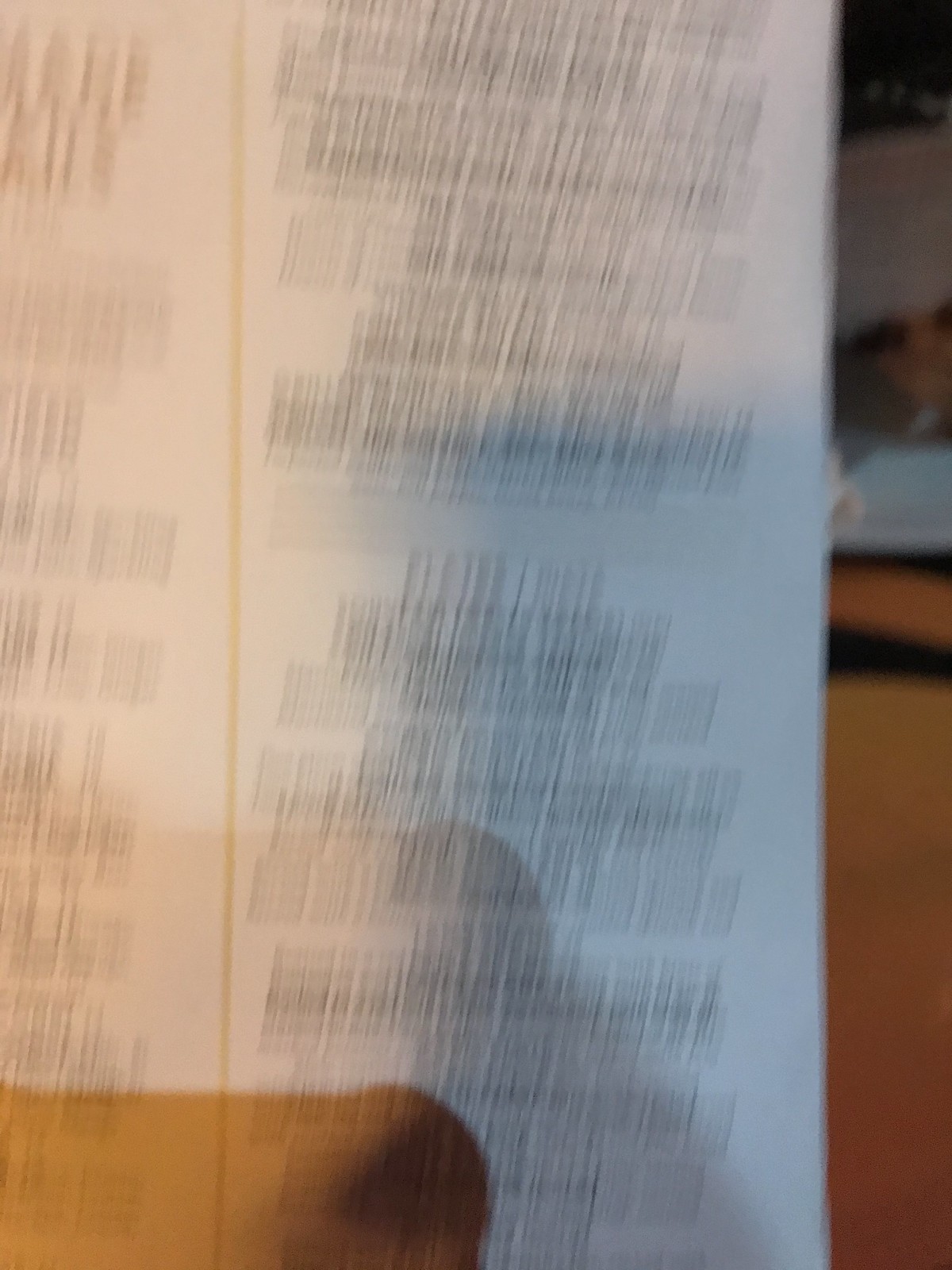The image is a rectangular portrait showing an extremely blurry white sheet of paper that occupies the majority of the frame. The paper stretches from the top to the bottom of the image and extends roughly 80% of the way from the left edge to the right edge, leaving a narrow background strip on the right. The paper is filled with many lines of black, seemingly all-caps text, but the blur makes the content unreadable. A prominent light yellow line runs vertically about two-thirds of the way from the left edge, positioned slightly to the left of the white paper. The top, left, and bottom edges of the paper are cut off, only the full right edge is visible. The lower left corner shows a tan or light brown area that appears to overlay the white paper. This section, covering the bottom 60% of the remaining image, and possibly resembling a table surface, extends upwards until the top right corner where black patches and a white segment are also visible. The overall impression is of a document, possibly a receipt or a menu, with complex textures and colors around it.